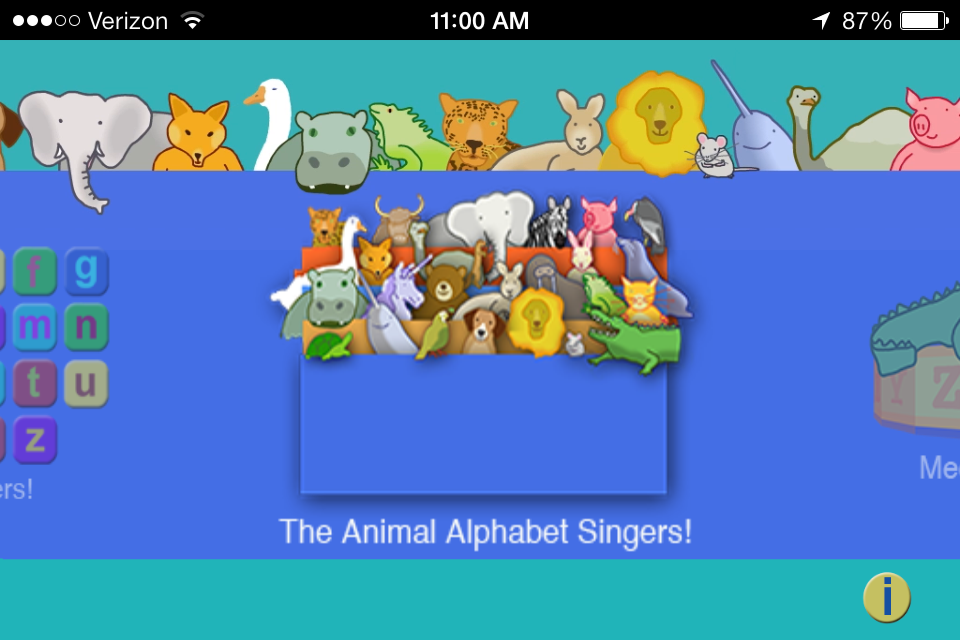The image captures a vibrant and colorful screen from a tablet or a cell phone. The top of the screen features a thin dark band that contains several key elements: on the left side, there are three solid white dots and three open dots, indicating a sequence of three out of five. Next to this is the word "Verizon" in white letters, alongside a weak signal strength icon. Centrally positioned in the dark band is the time, showing "11 a.m." To the right, an information icon displays the battery level at 87% along with the battery icon.

Below the dark band, the main page of the screen is highly colorful. A teal-colored band stretches across the top, embellished with several simple drawings of animals. From left to right, the animals depicted are a gray elephant, a fox, a goose, a hippo, an iguana, a leopard, a rabbit, a lion, a mouse, a shark, an ostrich, and a pig, each illustrated in different hues.

The central portion of the screen is predominantly purple, containing a segment of seven colored blocks arranged in two columns on the left side. The first column has four blocks labeled F, M, T, and Z; while the second column has three blocks labeled G, N, and U. The blocks are in various bright colors.

Within this purple section, there's also a prominent blue rectangular box displaying a collection of the same animal drawings found on the teal band at the top, along with additional animals. Beneath this blue rectangle, there is text in white which reads, "The Animal Alphabet Singer!" On the right side of this text, a partially visible image appears to be an alligator tail positioned above a block with the letter Z.

The bottom of the screen features another teal band, inside which, on the bottom right corner, is a grey circle with a blue eye symbol, likely representing an information button.